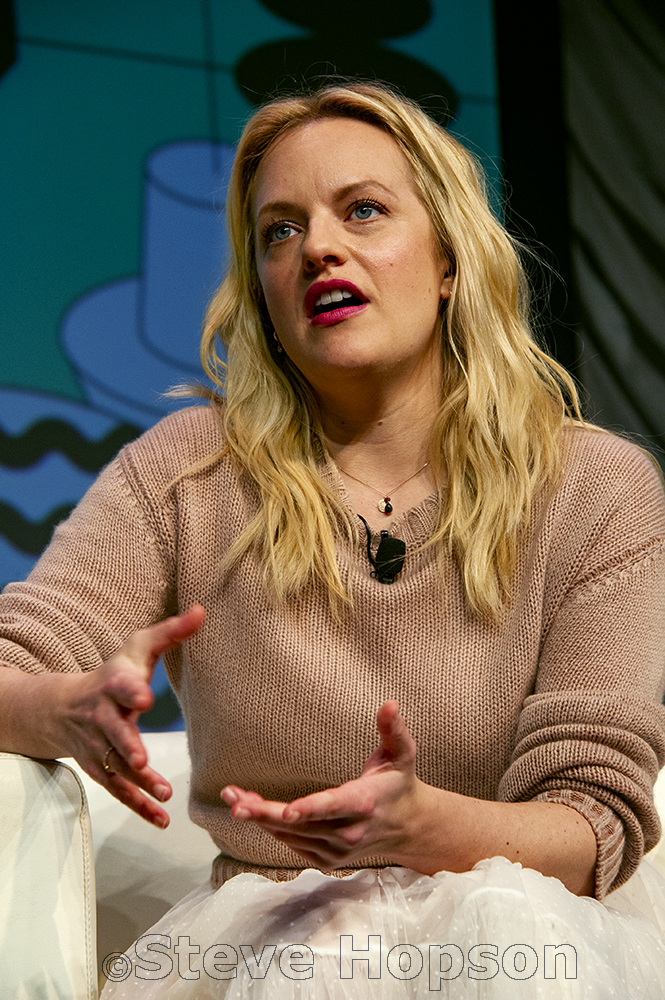The photograph features a woman visible from the waist up, seated in a white leather armchair. She has long blonde hair that falls to chest level on both sides. The woman is wearing a white skirt and a peach-colored long-sleeve sweater, with the sleeves pulled back to her elbows. Attached to the collar of her sweater is a black lapel microphone, and she wears a gold chain necklace with a small black and white pendant. The woman is facing slightly forward and towards the top left corner of the image, her mouth open as if speaking, and her hands are gesturing mid-speech. Her right arm rests on the arm of the chair, while her left arm is positioned on her lap. The backdrop reveals a wall with various drawings, including a hat and some designs on the left, and green and black lines on the right. At the very bottom of the photograph, there's a watermark in clear lettering that reads, "Copyright Steve Hopson." The overall scene suggests the woman is engaging in a conversation or possibly an interview, marking her as a notable figure.